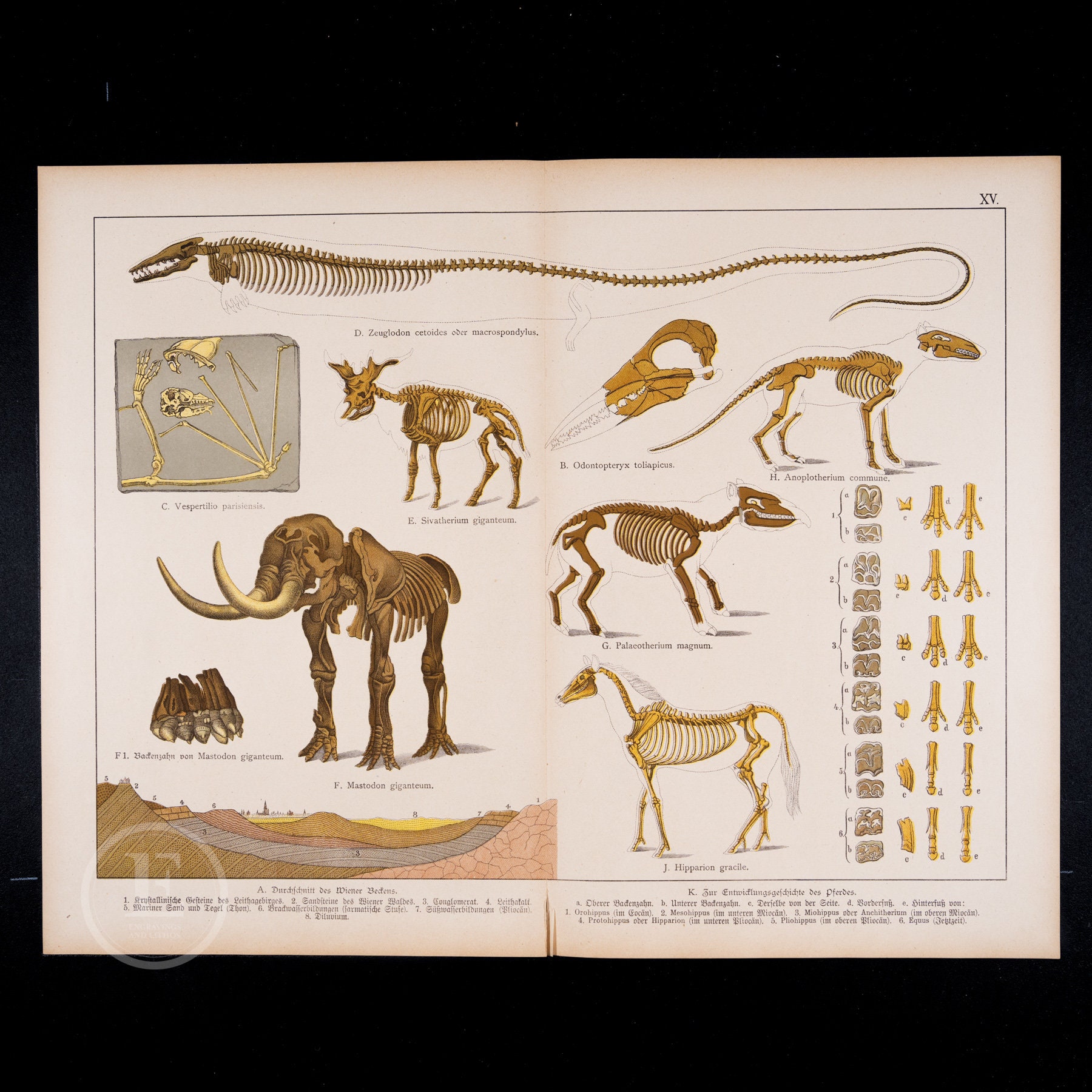In this image, an open book reveals two pages filled with detailed illustrations of various skeletons from different species, both prehistoric and modern. On the left page, there is a detailed depiction of what appears to be the skeleton of either a woolly mammoth or a mastodon, characterized by its large tusks and robust build. Additionally, there is a skeleton that closely resembles that of a modern-day horse, showcasing its distinct equine features. Among the prehistoric specimens, there are also skeletal structures that look like those of dinosaurs or large lizard-like creatures, complete with elongated limbs and tails.

On the right page, more skeletons are illustrated, including what appears to be a creature with an elongated heel, giving a unique insight into its skeletal anatomy. Both pages feature diagrams of various skeletal feet, providing a closer look at the distinctive bone structures of the animals depicted. The images dominate the pages, with minimal text present at the bottom, serving as brief labels or explanations.

The background of the image is entirely black, making the details of the book stand out prominently. In the bottom left-hand corner of the image, there is a watermark consisting of a capital letter "E" enclosed in a circle, subtly indicating the source or ownership of the image.